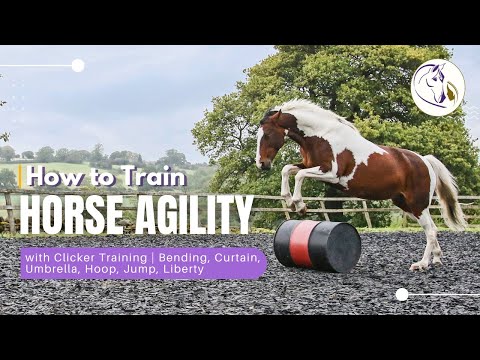This image features a black and white horse, distinguished by black splotches and a white blaze down its face, majestically leaping over a black and white pole. The hurdle is set against two bright blue trapezoidal stands and supported underneath by several brown boxes. The dynamic scene unfolds within an outdoor ring, encircled by a rustic wooden fence, backed by a grassy hill and a large tree stretching skyward. A woman with a ponytail of brown hair, clad in a dark blue vest over a long-sleeve shirt and black pants, runs energetically behind the horse. At the bottom of the picture, text reads "Horse Agility Training: How to Use Clicker Training for Horse Agility," accompanied by a small circular logo depicting a horse.